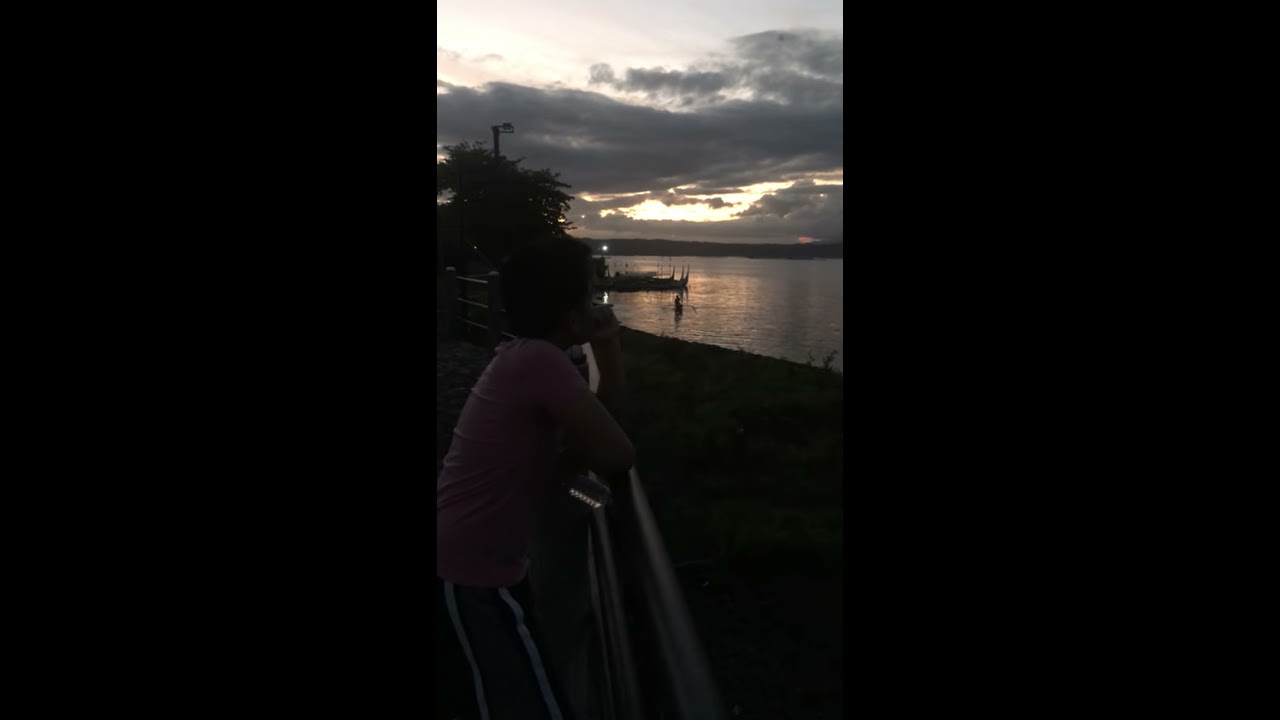The image, likely a screenshot from a video given its vertical format with black borders, shows a dimly lit scene probably taken around sunset or perhaps just after or before. The focal point is a person, possibly female and wearing glasses, leaning on a silver metal fence. She has a purple shirt and black pants with white stripes. Standing next to her is another figure dressed in striped shorts and a blue shirt, both gazing out towards a serene body of water. The landscape features a grassy patch near their feet, leading to a wide expanse of water. Beyond the water stretches a strip of land. The sky is painted with dramatic strato-cumulus clouds, with the sun obscured either behind these clouds or positioned just outside the frame. There's a solitary tree in the distance, and a dock is visible as well, adding depth to the tranquil, moody scene.